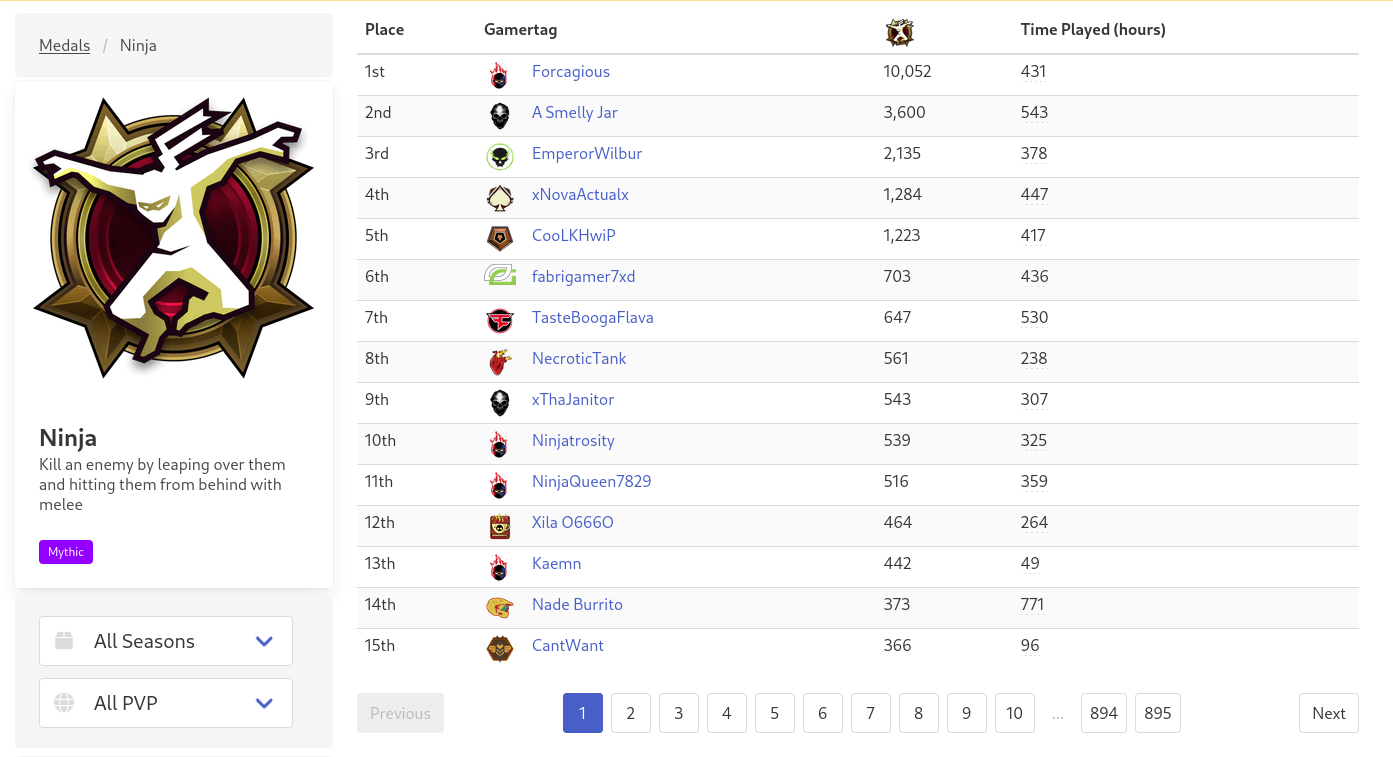This image displays detailed rankings and playtimes from a video game leaderboard. On the left, the section highlights a character titled "Metal Slash Ninja," featuring an illustration of a ninja clad in white, set against a background resembling a throwing star. Below this image, there is a description reading: "Ninja - Kill an enemy by leaping over them and hitting them from behind with melee." A small purple box with the word "Mythic" is present, and beneath it, there are dropdown menus labeled "All Seasons" and "All PvP (Player vs Player)."

On the right side of the image, the leaderboard is displayed with columns for player rankings, gamer tags, points indicated by a ninja icon, and total playtimes in hours. The rankings are as follows:

1. **Furgacious:** 10,052 points, 431 hours played
2. **A Smelly Jar:** 3,600 points, 543 hours played
3. **Emperor Wilbur:** 2,135 points, 370 hours played
4. **Six Novet, Actual X:** 1,284 points, 447 hours played
5. **Cool LKHWIP:** 1,223 points, 417 hours played
6. **Fabregamer7xd:** 703 points, 536 hours played
7. **Taste Bugha Flava:** 647 points, 537 hours played
8. **Necrotic Tank:** 561 points, 238 hours played
9. **X the Janitor:** 543 points, 307 hours played
10. **Ninjurocity:** 539 points, 325 hours played
11. **Ninja Queen7829:** 516 points, 359 hours played
12. **Xzilla0666:** 464 points, 264 hours played
13. **KM:** 442 points, 49 hours played
14. **Nade Burrito:** 373 points, 771 hours played
15. **Can't Want:** 366 points, 96 hours played

The leaderboard is noted as being on the first of 895 pages, with a button available to navigate to the next page.